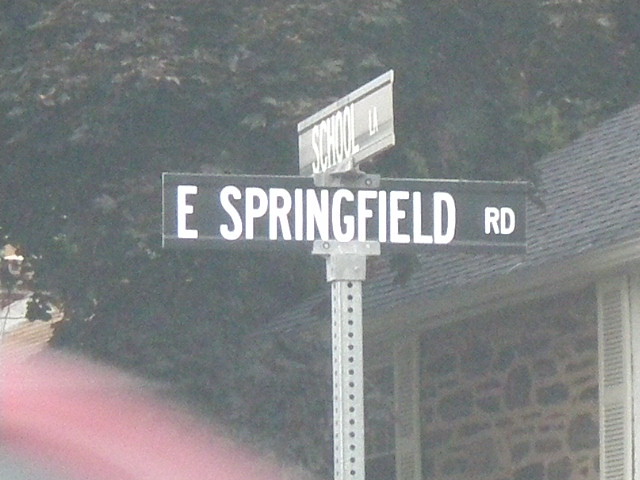This image depicts a street sign positioned at the intersection of East Springfield Road and School Lane. The signpost indicates that School Lane runs perpendicular to East Springfield Road. The photograph appears to have been taken from inside a car, as evidenced by the slight blurriness and haze likely caused by the windshield. The image quality is somewhat compromised, possibly due to cropping or zooming in on the original photo.

In the background, there is a brick house, although it may be constructed with faux brick. The house is partially obscured, with only the corner and roof visible. A large, dark green tree with a full canopy looms over the house, adding a lush, natural element to the scene. The perspective of the shot suggests the photographer was seated in the car, capturing this everyday moment from a dynamic angle.